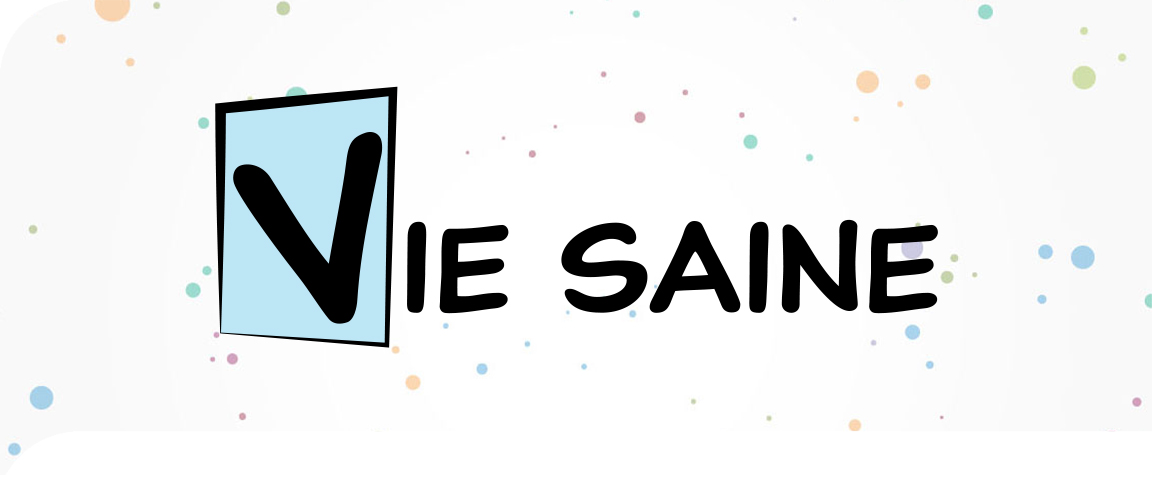The image features a central, prominent logo with the word "VISAYNE" in bold, black, all-capital letters. The initial "V" is notably highlighted in a blue square with a black border. The background is predominantly off-white and sprinkled with various multicolored dots and circles—ranging from orange, red, green, blue, to purple—creating a bubble-like pattern. This vibrant and colorful design is presented in a rectangular banner style, making it resemble a potential logo or business card header, perfectly centered to draw attention.